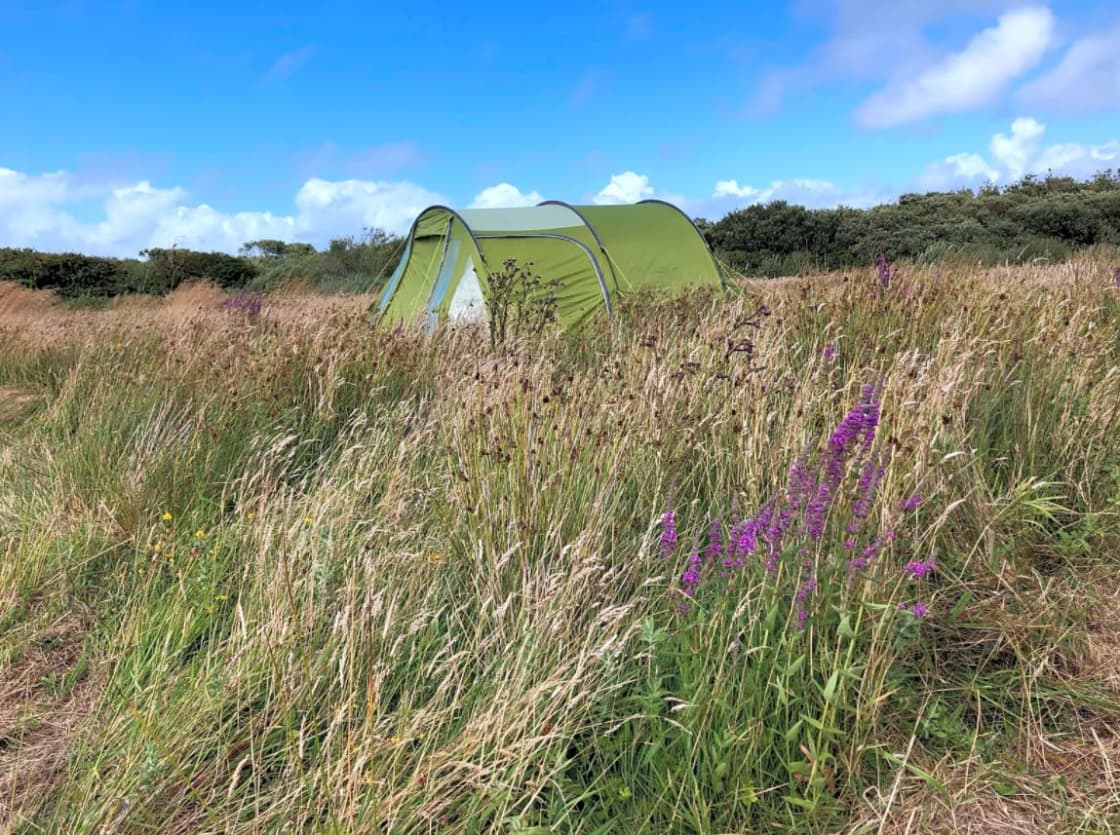In the center of this vivid photo, a pale green, dome-shaped tent stands amidst a sprawling field of tall, varied grasses and wildflowers. The high grasses partially obscure the tent, indicating it is firmly set in the middle of this natural expanse. The field is vibrant with different colors; purple wildflowers grace the foreground, while small yellow blooms and a mix of green, white, and brown grasses add texture. Some of the grasses appear dried and dead, adding to the field's rustic charm. The bright blue sky, dotted with white clouds, enhances the serene atmosphere, and a line of trees and shrubs forms a natural border in the background. The tent, zipped up completely, shows no sign of human presence or additional camping gear, suggesting a secluded, minimalist camping spot in the midst of this picturesque landscape.